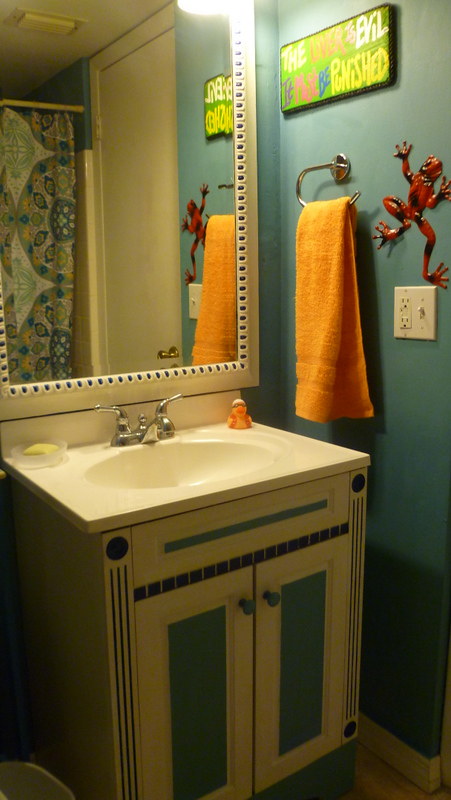The bathroom is painted in a soothing blue hue and features a single vanity primarily occupied by a sink, leaving minimal counter space. On the counter, there is a playful rubber duck and a soap dispenser. The vanity is equipped with basic silver chrome fixtures. Behind the vanity is an expansive mirror that enhances the room's brightness. Beside the mirror, an orange towel hangs from a silver chrome bar affixed to the wall. Above the light switch panel, there is a whimsical frog art piece. Additionally, another green art piece with text is displayed, adding a touch of personality to the space.